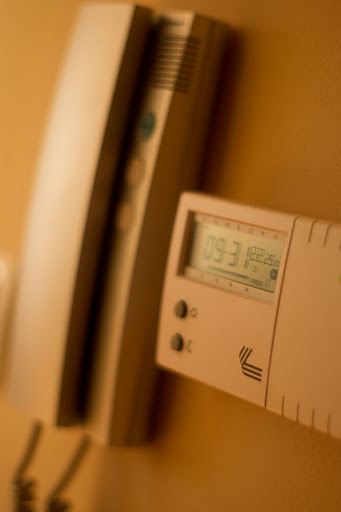This image features a slightly blurry close-up of a digital clock mounted on a mustard-colored wall, next to a modern landline telephone. The clock is rectangular and encased in light cream-colored plastic. Its display reads "9:31:22", flanked by two buttons below it. One button has a sun symbol, indicating perhaps a daytime setting, and the other has a crescent moon symbol, likely for nighttime settings. A small logo with three black stripes turned up like a ribbon is positioned beneath the display. Beside the clock is a sleek, rectangular cream-colored landline phone with sharp edges and a slim receiver. The setup casts distinct shadows on the wall, adding depth to the scene.